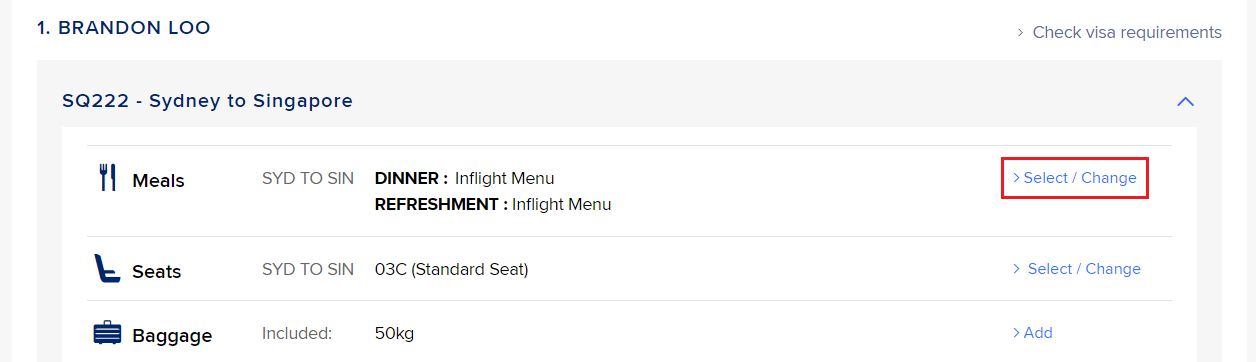This small rectangular photo contains detailed travel information formatted in a clear way. At the top left, the number "1." appears, followed by the name "Brandon Blue" in uppercase dark blue text. On the top right, there is gray text that reads "Check Visa Requirements."

Beneath this top section, there's a dark blue line of text that states "SQ222 – Sydney to Singapore" on the left side. Below this line, three categories are displayed in black uppercase with corresponding details:

1. **Meals:** Displayed as "SYD to SIN Dinner" underlined by "In-flight menu dinner and refreshment" in lighter lowercase gray text.
2. **Seats:** Listed as "SYD to SIN 03C Standard Seat."
3. **Baggage:** Indicated as "Baggage included: 50 kg."

Each of these sections has an interactive element on the right side. For Meals and Seats, there is blue text "Select/Change" outlined with a red rectangle, and for Baggage, the blue text "Add."